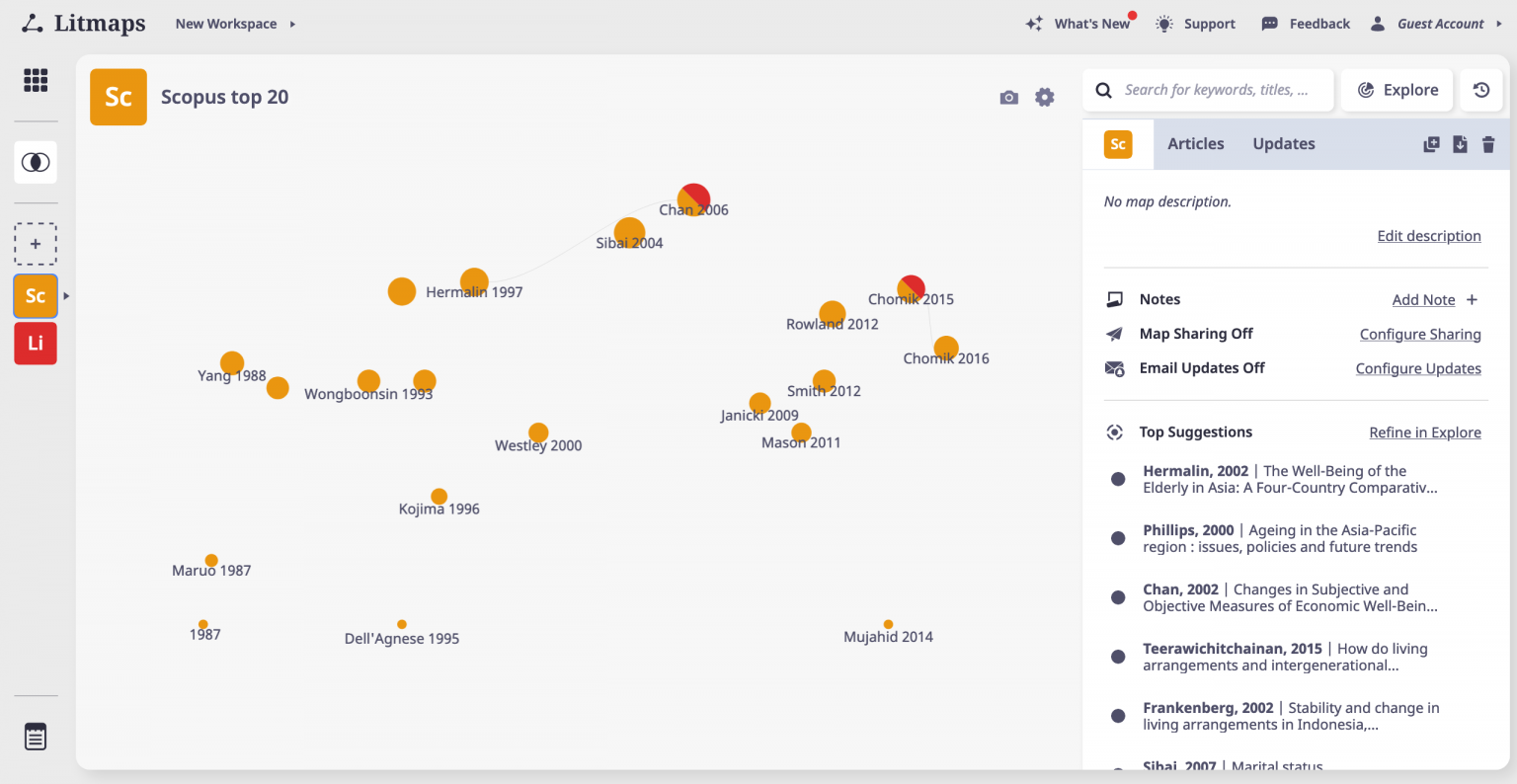A screenshot of the Lit Maps website is bordered by gray bars, featuring a vertical menu on the left and a horizontal menu at the top. In the upper left corner, a black icon composed of three circles and a triangle connected by lines is visible. Adjacent to this icon, the site title "Lit Maps" is displayed in black font. Next to the title, there is a drop-down menu labeled "New Workspace."

On the right side of the horizontal menu, a series of icons and labels appears: a three-star icon followed by the text "What's New," a lightbulb icon with the text "Support," a chat bubble icon with the text "Feedback," and a human silhouette icon with the text "Guest Account."

The left vertical menu includes several distinct symbols. From top to bottom, these are: an array of three black dots in three lines, a white square with two black circles inside it, a square formed by small dots, an orange square with white letters "SC," and a red square labeled "Li."

The main screen on the right side of the webpage prominently displays "Scopus Top 20" at the top.